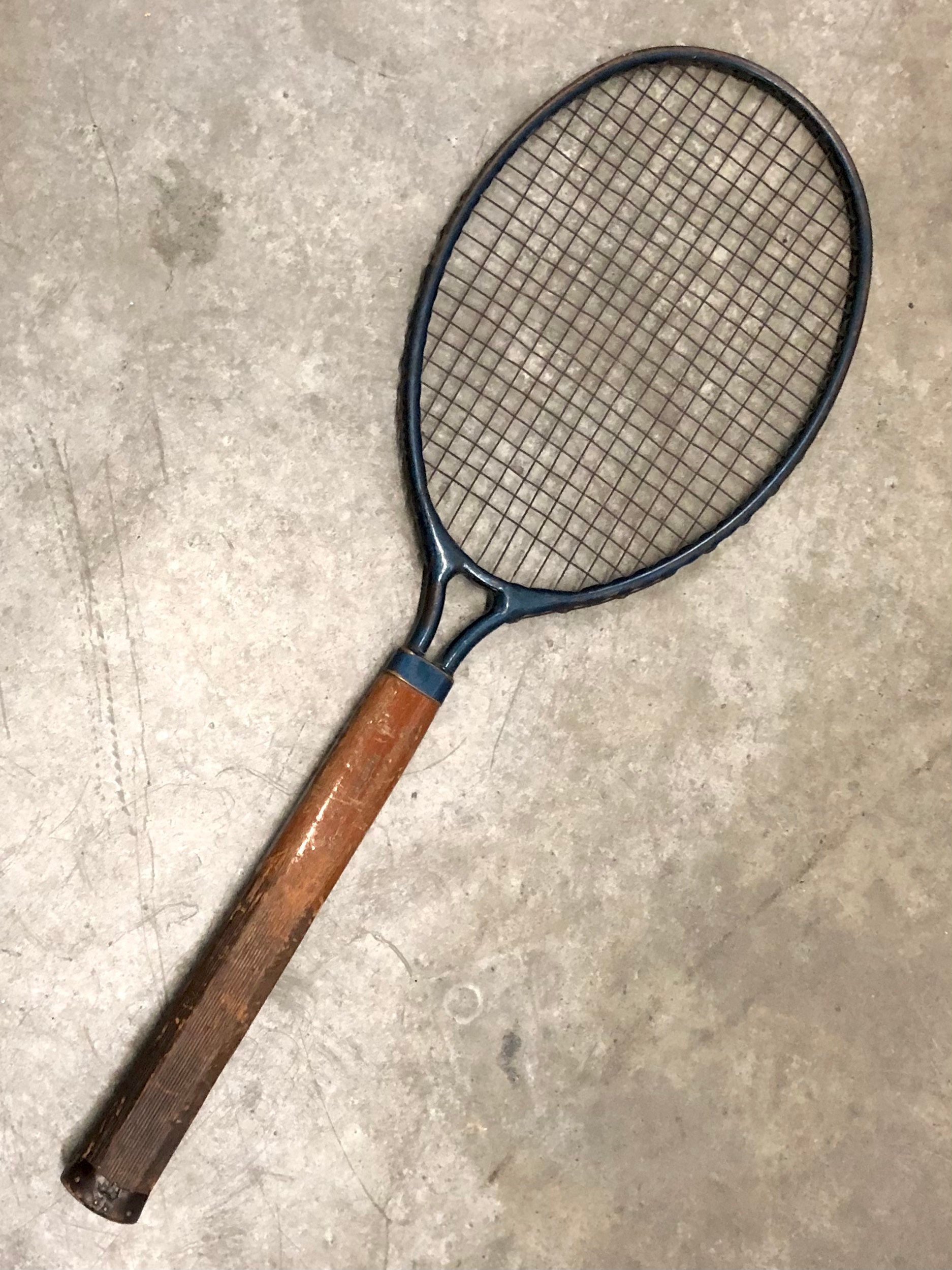The image displays a vintage tennis racket resting on a worn, stained concrete floor. The racket's handle, located on the left, stretches diagonally towards the right and is crafted from dark brown wood that appears cracked and weathered, indicative of its age. The frame of the racket is black, while the netting comprises black strings. The backdrop consists of a rough, patchy stone floor, showcasing an array of cream, brown, and greenish-gray hues, with prominent lines, stains, and pits. The aged and well-used condition of both the racket and the floor highlights their lengthy history, giving the overall scene an antique and rugged appearance.